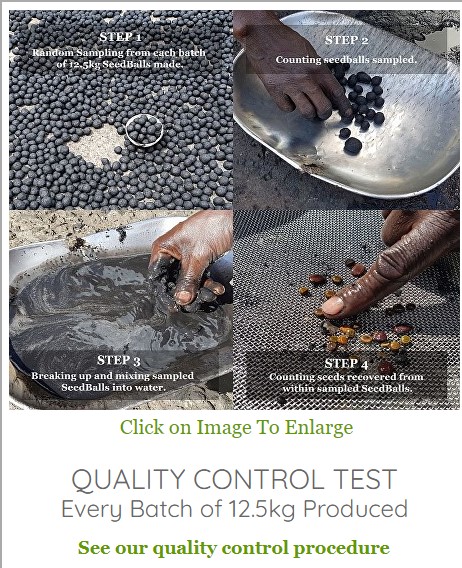This image illustrates the detailed steps involved in performing a quality control test on seed balls. 

1. **Random Sampling**: The first step displays a selection of seed balls from a larger batch, emphasizing the necessity of obtaining a random sample.
  
2. **Counting Seed Balls**: In the second step, the image shows a silver pan with the sampled seed balls, where the next action involves counting the number of seed balls collected.

3. **Breaking and Mixing**: The third step features the same silver pan, now with the sampled seed balls being crushed and mixed into water. This process turns the water black, indicating thorough mixing.

4. **Seed Recovery**: The fourth and final step displays the seeds extracted from the seed balls, spread out over a mesh strainer. This step focuses on cleaning the seeds by removing any remaining black residue.

Each batch subjected to this quality control procedure weighs 12.5 kilograms, ensuring consistency in the production process.